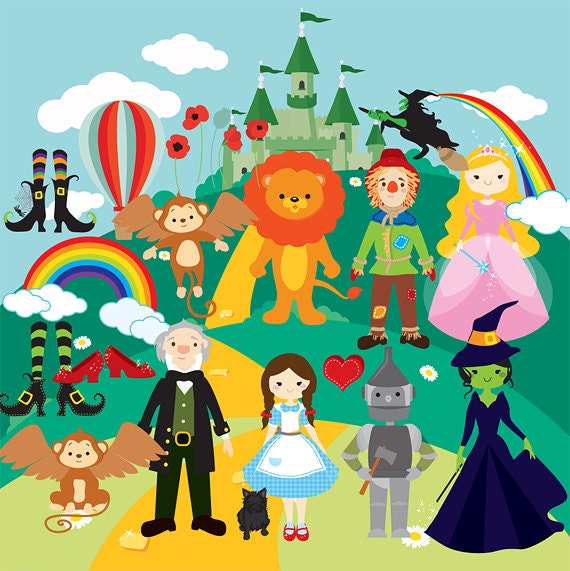The image is a colorful, two-dimensional clip art-style illustration of the Wizard of Oz with a whimsical and child-friendly flair. Featured prominently in the background is the iconic Emerald City castle, done in shades of green. A green-skinned witch in a black outfit flies on a broomstick towards the castle, with a vibrant rainbow trailing from the tip of her hat. Clustered around the scene are various characters from the classic tale: a smiling Dorothy, with her brown hair in braids and wearing a blue gingham dress and white apron, stands beside Toto. The Tin Man, depicted in various shades of grey and with a funnel on his head, holds an axe. The Cowardly Lion and the Scarecrow are also present, each rendered in a cutesy, friendly manner.

Additional figures include a fairy godmother-like rendition of Glenda the Good Witch, adorned in a pink dress, a blue wand with a star, yellow hair, and a pink tiara. An older gentleman in a black suit and green vest is also part of the ensemble, likely the Wizard. There are playful flying monkeys with brown fur and wings, one of which is charmingly sitting and gazing at a daisy. Red poppies, symbolizing the fields from the story, are scattered throughout, and several pairs of shoes, including striped witch’s stockings and boots and shiny ruby red slippers, add to the visual storytelling. Above, rainbows and clouds, along with a red and blue hot air balloon, complete the lively and magical scene. Overall, the illustration is a delightful and vivid tribute to the beloved characters and settings of the Wizard of Oz.